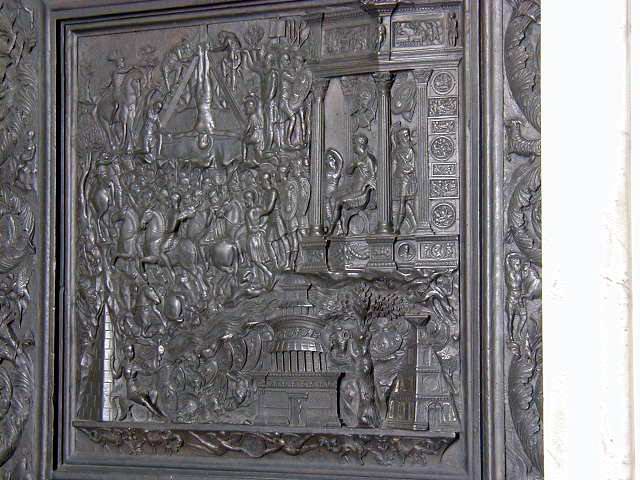The image depicts an intricately carved, grayish to grayish-brown metal plaque or art object, rectangular in shape and possibly taken indoors with a portion on the left appearing whited out, potentially indicating the edge of a doorway. The plaque showcases an elaborate 3D relief pattern, framed with a "square within a square" design. The central scene is vivid with historical and dramatic elements. It features a bustling crowd, reminiscent of an ancient Roman setting, filled with soldiers, horses, carriages pulled by two horses, and various buildings, including a three-tiered tower, pyramid-shaped temples, and classical pillars dripping with vinage. Notably, a disturbingly detailed figure hangs upside down by their feet, arms outstretched in a crucifix-like pose, amidst this tumultuous gathering. Surrounding this central figure are more caricatures of Roman life—people conversing on a balcony, dancers, architectural detailing resembling roots intertwining with animals, and lush trees. This complex composition captures a moment rich with historical allusion and artistic depth.